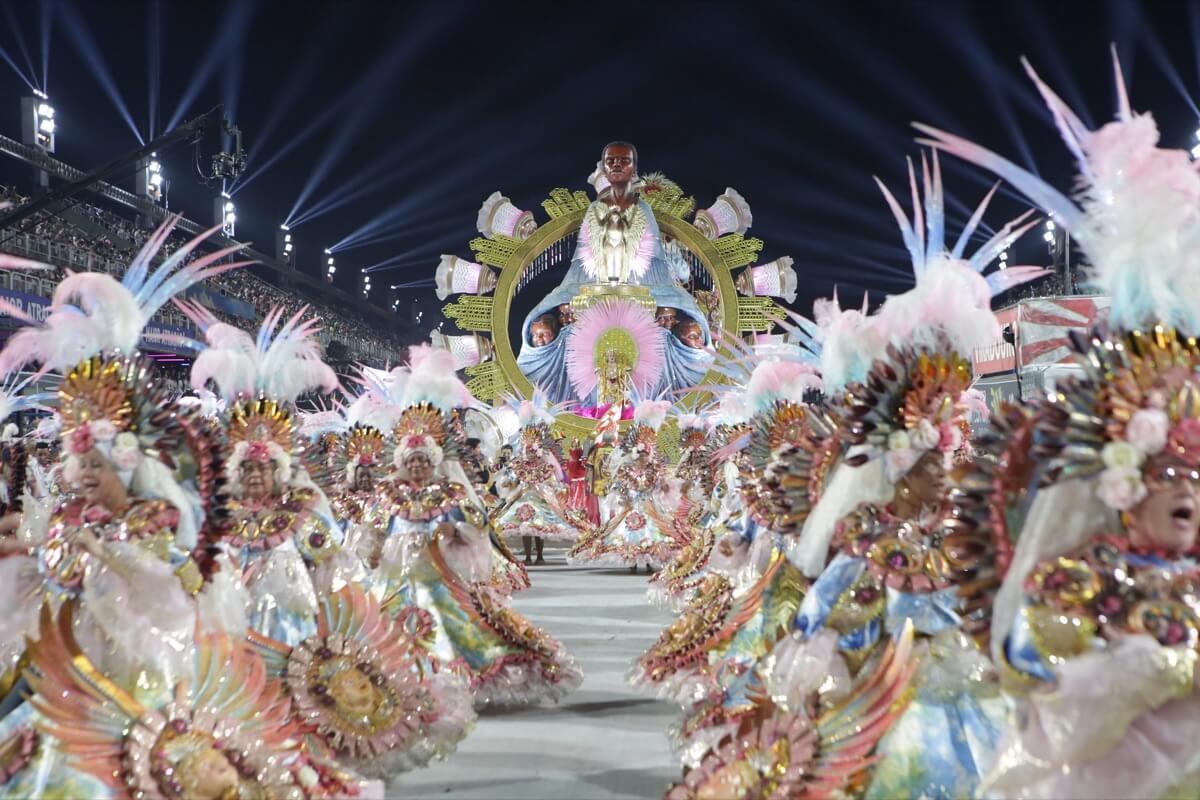This high-quality photograph captures the vibrant essence of a Rio de Janeiro Carnival parade, illuminated against the deep midnight blue of the night sky. The scene is bustling with an array of dancers adorned in elaborate costumes that exude a cotton candy charm through their soft pink, light blue, gold, and white hues. Each dancer is topped with a grand headdress featuring golden and silver feathers, flowers, and intricate crowns, adding to the festivity's opulence.

The performers, a mix of older men and women, are festooned in flowing white robes embellished with cherubic motifs surrounded by gems and feathers, evoking a celestial theme. They move in coordinated lines, dancing and celebrating with palpable joy, reflected in the throngs of spectators lining the stadium stands on either side of the street.

Dominating the center of this captivating scene is an ornate float. This float features a round gold structure, reminiscent of Mayan architecture, and is crowned with an image of a man dressed in a pristine white suit and tie. Accompanying this central figure, a cherub's face encircled in decorative elements, complements the grandeur of the parade. The detailed display, along with the jubilant dancers and the festive atmosphere, encapsulates the essence of this magnificent cultural celebration.